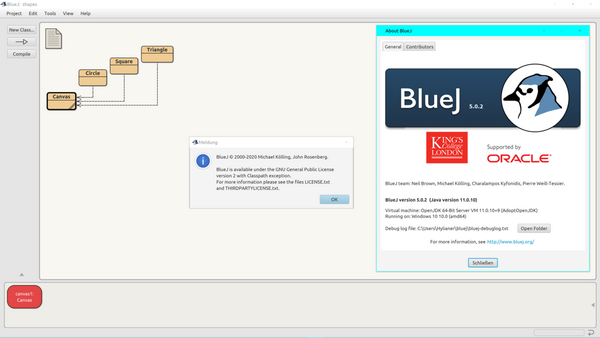The image is a screenshot of a web-based builder interface. At the center of the screen, there is an obscured dialogue or information box. This box's header features a blue circle with a lowercase "i" in the middle, indicating information or help. At the bottom right of this box, there is a lighter blue button that appears to be labeled "OK." 

To the right of the dialogue box, the text "BlueJ 5.0.2" is visible, suggesting the software version. Below this, "King's College London" is displayed next to a red box. Adjacent to this is the text "supported by Oracle." 

In the top-left corner of the screen, there is a graphical element composed of four interconnected boxes: three on top leading to a single box below, possibly indicating a hierarchical structure or navigation path.